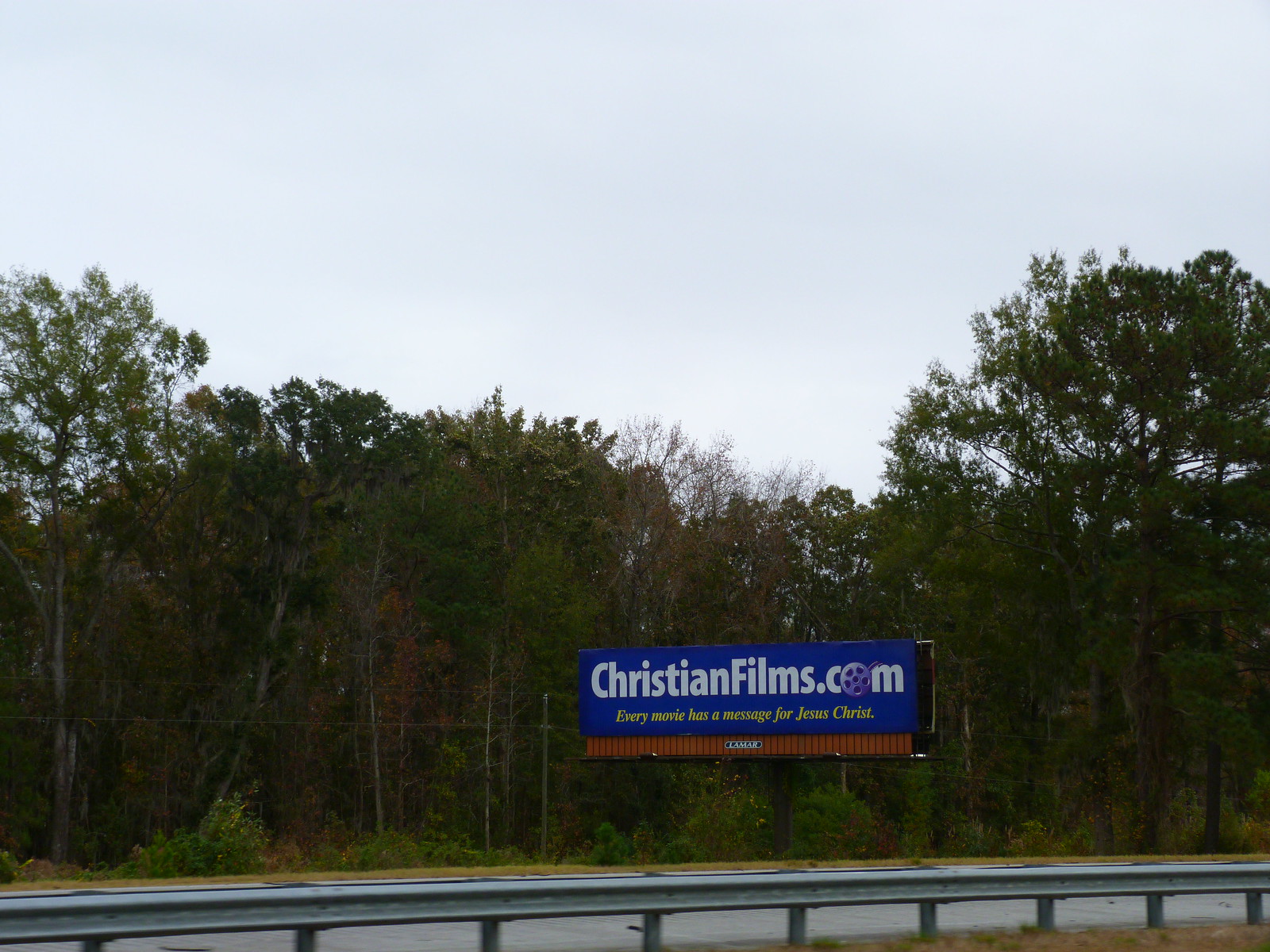The photograph captures a silver steel guardrail spanning horizontally across the bottom of the frame. Just beyond the guardrail, a strip of pavement hints at a highway partially obscured by the guardrail itself. The background reveals a densely populated forest with dark green and brownish rust-colored leaves, giving a rich texture to the scene. Amidst the trees stands a prominent blue and red billboard. The top of the billboard is primarily blue with the text "christianfilms.com" in white, where the 'O' in '.com' is artistically designed as a movie reel. Beneath this, in yellow text, the slogan reads, "Every Movie Has a Message for Jesus Christ." The bottom section of the billboard is red. Above the treetops, the sky is a very hazy white, devoid of visible sun, clouds, or blue hues, adding a serene yet muted backdrop to the vibrant billboard and the verdant forest.